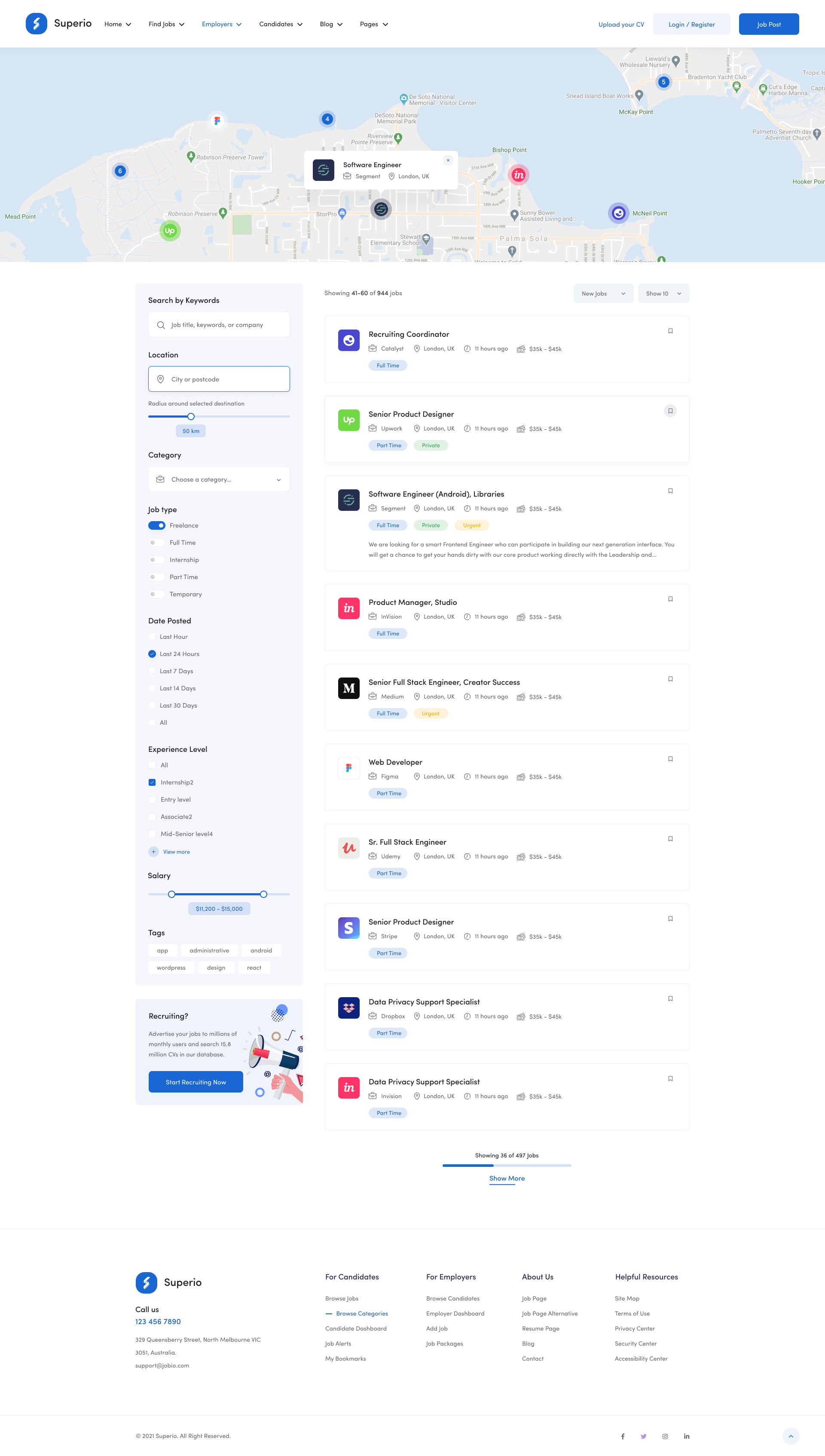This image depicts the homepage of the Super.io website. In the top left corner, the Super.io logo is prominently displayed, featuring a white "S" within a blue circle. Moving rightward across the top navigation bar, there are tabs labeled "Home," "Find Jobs," "Blog," "Login," and "Register." Additionally, there is an option for "Job Postings."

Below the header, a map is shown prominently in the center of the page. On the left sidebar, there is a search functionality with various filtering options, including search by keywords, category, location, job type, experience level, and salary range. There's also a section for tags at the bottom of this sidebar.

The main section of the page features a list of job results generated by the search, displayed in a vertical column. At the bottom of the job listings, there is a "Show More" button, allowing users to load additional job results.